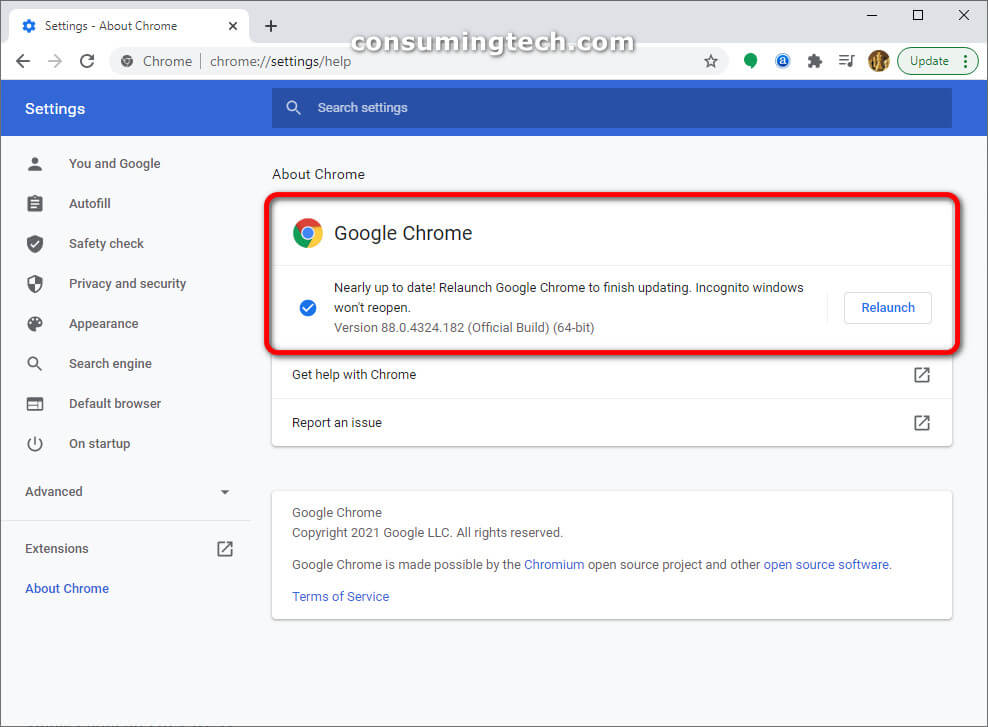### Detailed Descriptive Caption:

The image features a digital interface with a light grayish-blue background bordered by a thin black line. In the top-left corner, a small white tab is prominently popped up, featuring a blue "settings" icon. To the right of this icon, the text "Settings - About Chrome" appears in black, followed by an "X" symbol at the end of the tab. 

Adjacent to this, within the blue border, there is another "X" symbol rendered in black. On the same blue border but to the far right, another "X" is present, followed by a square icon and a dash which boldly displays "ConsumingTech.com" in white. Directly below this, there is a search bar flanked by four icons, and a profile picture appears to the far right. Next to the profile picture, there is a blue tab labeled "Update."

Further down, a blue border spans the width of the page. On the left side of this border, the word "Settings" appears in white text. About two inches to the right, there is a search tab that extends all the way to the right side of the screen, containing the text "Search settings."

Underneath the blue border and back on the light grayish-blue background, there are eight icons aligned vertically on the left side, each corresponding to a setting category. The first icon represents a profile, labeled "You and Google." There are six such icons in total, and beneath the sixth icon, the text "Advanced" appears with a dropdown tab on the right side. 

Below the "Advanced" section, there is an "Extensions" section with a small square icon featuring an arrow pointing up and to the right. Following this, "About Chrome" is highlighted in blue text. 

Beneath the "Search settings" label, which appears in black, the "About Chrome" section is detailed within a large rectangle with a red border. Inside this rectangle, the Google Chrome icon is displayed, followed by the label "Google Chrome" to the right. Below this, a thin line is underlined, beneath which a blue circle with a white checkmark contains two lines of black text. Further down, the version number of Chrome is specified, with a white tab highlighted in blue that says "Relaunch."

Additional options listed below this section include "Get help with Chrome" and "Report an issue," both in white text. More detailed information about Google Chrome, including dates and other relevant data, follows these options.